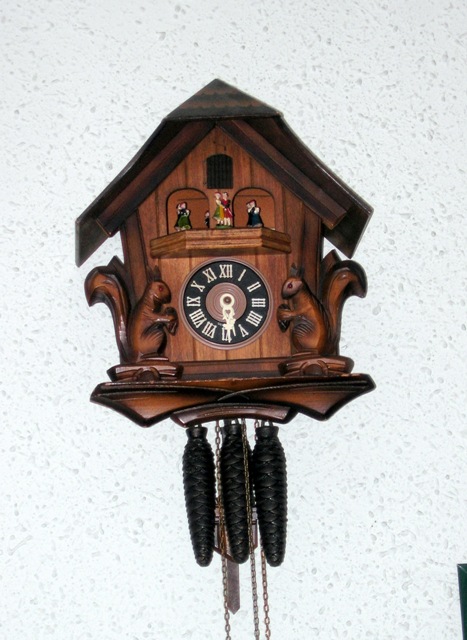The photograph showcases a vintage wooden cuckoo clock designed to resemble a house intricately carved from chestnut-colored wood. Dominating the center is a black circular clock face adorned with white Roman numerals and reflective silver metal hands. Flanking the clock face are detailed carvings of squirrels holding acorns, positioned symmetrically on either side and facing each other.

Above the clock face, a small carousel with multiple dancing couples is visible, and crowning the structure is a little door with a rounded top. The roof, distinctively darker than the rest of the clock, adds to its charming old-fashioned appeal. Hanging below the clock housing are three weight chains resembling long black pine cones, further emphasizing its traditional design. The entire antique clock is mounted on a white, speckled, textured wall.